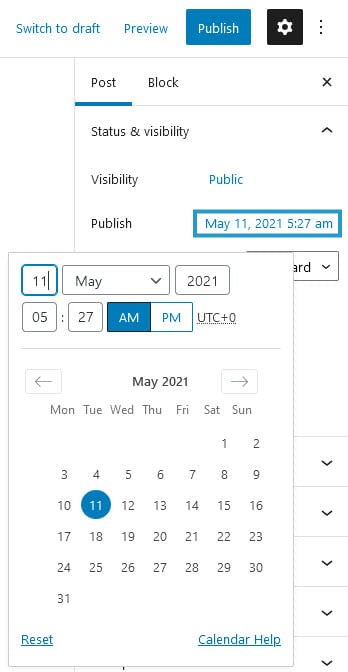A pop-up interface is displayed featuring a white rectangular dialog box bordered in gray. The top section contains several input fields:

1. **Outline Field:** Contains a box outlined in teal, displaying the number "11" in black.
2. **Month and Year:** Adjacent fields display "May" and "2011" respectively.
3. **Time and Date Fields:** 
    - One field says "05", followed by a colon and "27."
    - A blue box, which is currently selected, displays "AM."
    - Next to it, there's "UTC+0" in black.

A thin gray line separates these fields from a mini calendar view of May. The calendar shows the abbreviations of the days of the week (MON, TUE, WED, THU, FRI, SAT, SUN). The first day of the month, May 1st, starts on a Saturday. All numbers in the calendar are displayed in black, except for the 11th, which is highlighted white with a teal circle around it.

At the bottom of the calendar, there are two options: "Reset" (underlined in blue) and "Calendar Help" (also underlined).

In the overlay behind this, at the top, the word "Post" is displayed in black and underlined in blue. Below, the section labeled "Status and Visibility" includes the following details:
- "Public" in blue under visibility.
- A line reading "Publish" in black.
- Date and time details in teal displaying "May 11th, 2021 at 05:27 AM," encased in a teal box.

Adjacent to this is another overlay box, partly obscured, with visible letters "ARD."

At the very top, the interface gives options to "Switch to Draft" and "Preview." To the right, a white "Publish" button stands out against a teal background. Lastly, a black square with a white gear icon represents settings at the top right corner.